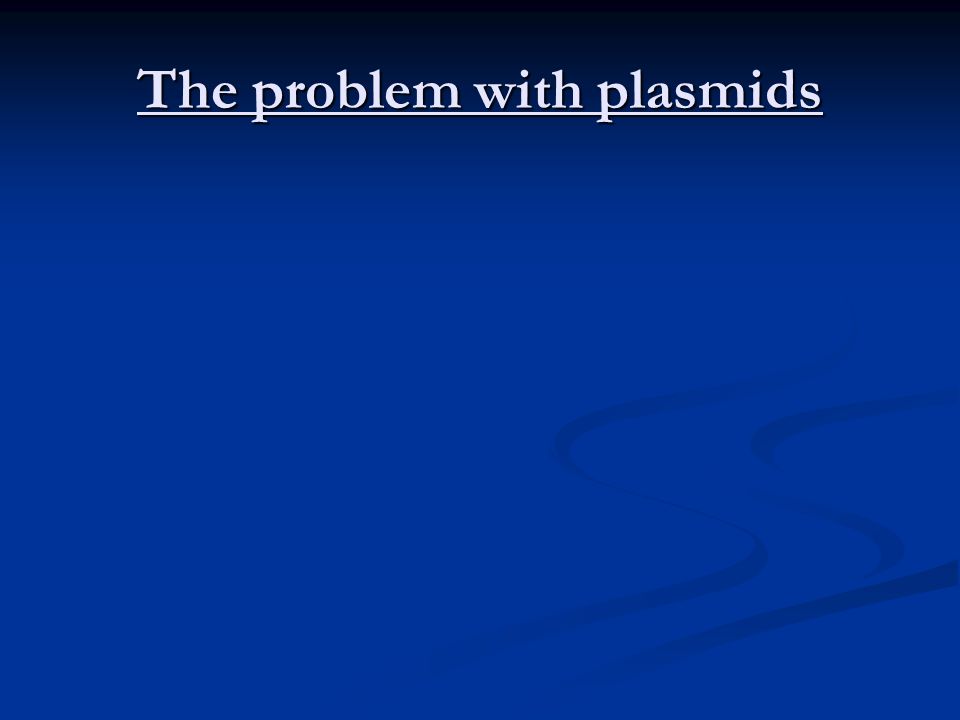This PowerPoint slide features a predominantly royal blue background with a strip of very dark blue, almost black, at the top. The background includes two wavy, S-shaped designs in a slightly darker shade of blue, originating from the bottom middle and curving towards the lower right of the slide. The slide is relatively minimalistic, containing just one line of white text centered near the top that reads "The Problem with Plasmids," with only the "T" in "The" being capitalized. This line of text is underlined in white. The overall impression is that of a title card or an introductory slide, characterized by its clean design and lack of additional content or bullet points.